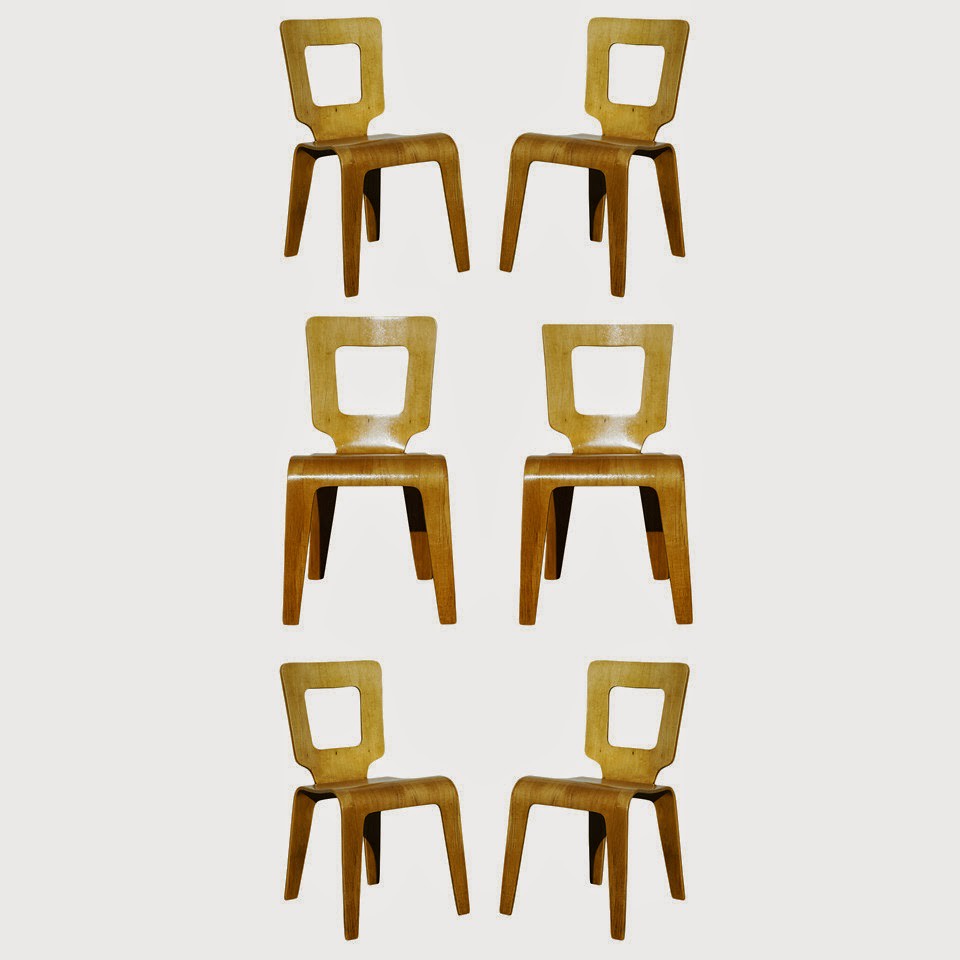The image presents a graphical representation of six identical, modern-style wooden chairs arranged in a vertically oriented, square format against an off-white, light grey background. Each pair of chairs is positioned in a distinct row; the top pair and bottom pair are angled inwards at 45 degrees facing each other, while the middle pair faces directly forward. The chairs are organized in a symmetrical grid: two chairs across and three chairs high.

All chairs share a polished finish and are designed with a stylish blend of materials: the seats and legs are a darker oak color, and the backrests are a lighter beech color. The backrests feature a distinctive cutout in the shape of a rounded-off square, providing a see-through element. The craftsmanship showcases artistically bent wood that curves to support both the seat and the back, highlighting the ergonomic design. The reflective surface of the wood adds a touch of elegance to the simplistic design, enhancing the overall visual appeal of the composition.